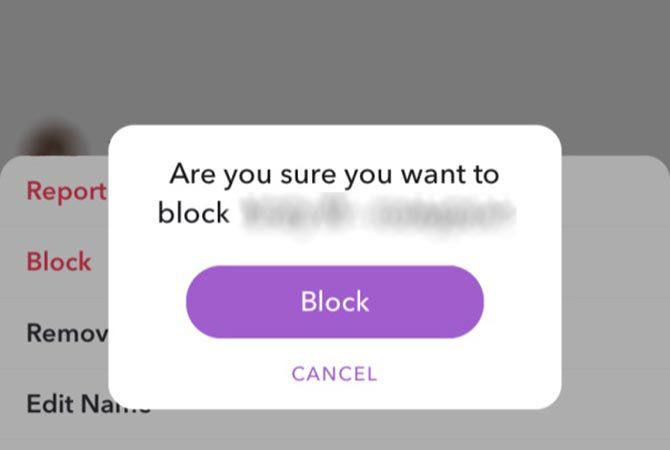In this image, we are viewing a user interface, likely from a social media application, displaying a partially obscured confirmation dialog. The dialog box prominently features a system message that reads, "Are you sure you want to block," followed by a name that has been intentionally blurred or blotted out. The central focus is a large purple button with the word "Block" written in white letters, indicating the action to permanently block the obscured user if clicked. Below this, there is a smaller option to "Cancel" the action, giving the user an alternative if they reconsider.

To the left of this dialogue box, partially visible red text displays “Report,” with the remaining text obscured. Below this, also in red, the word "Block" is visible, though further details are unreadable. Beneath these options, black text offers additional actions: "Remove" and "Edit Name," though the full extent of these options is also obstructed by the dialogue box in the center. The overall layout suggests a mechanism for managing social interactions and moderating content by blocking or reporting users, editing user details, or removing them from a list.